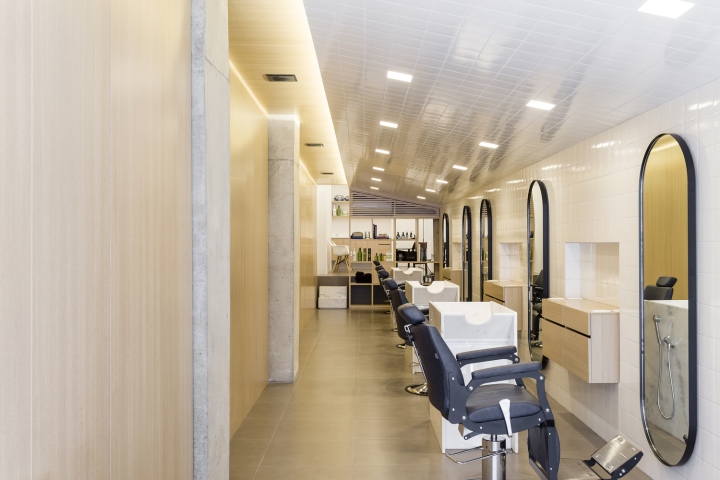The image depicts the interior of a modern, narrow hair salon. The salon features five black, high-backed, reclining chairs lined up along a very light-colored tiled wall, separated by white columns and light brown shelving. Each chair faces a long, oval mirror with a black frame, mounted on the wall. Adjacent to every chair is a small, white cabinet for salon supplies. The ceiling is covered in white tiles with small rectangular lights, illuminating the space and giving it a clean and bright appearance. Toward the back of the room, shelves stocked with various hair care products such as shampoos and conditioners are visible, adding to the organized and tidy look of the salon.